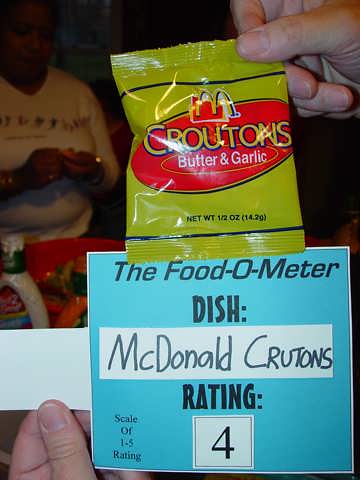In this indoor photograph, a pair of light-skinned hands prominently displays a yellow package labeled "Croutons" in bold yellow text, set against a red circle. The familiar McDonald's logo is also visible on the package. Below the word "Croutons," the package specifies "Butter and Garlic" in white text. Additional details include two black stripes and black text indicating the net weight as "1.5 ounces, 14.2 g."

Beneath the crouton package, a blue slip of paper is held, featuring black text that reads: "The Food-o-meter. Dish: McDonald's Croutons. Rating: 4. Scale of 1 to 5 rating."

In the dimly lit background, an indistinct figure is barely visible, creating a sense of depth. Also visible in the background are a bottle of salad dressing and what appears to be a red bowl, adding context to the photograph's setting.